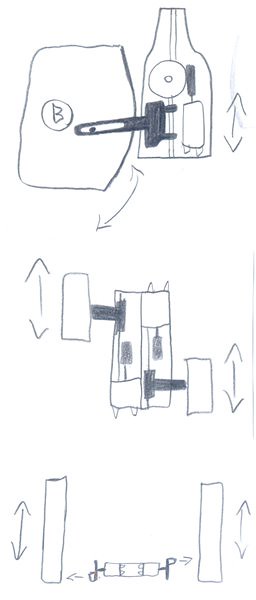This intricate pencil sketch on white paper appears to be a technical diagram, comprising three distinct segments arranged vertically and interconnected by arrows. 

The top segment depicts an apparatus resembling a bottle housing intricate gears. Extending from the bottle is a tool reaching towards an area labeled 'B.' 

The middle section portrays a broader rectangle filled with smaller squares and rectangles, connected via black bars to two additional rectangles positioned on either side. 

The bottom section features two elongated vertical bars flanking a horizontal bar. On either side of the horizontal bar are elements resembling the letter 'P', with arrows directing attention to the adjacent vertical bars. 

This detailed diagram seems to illustrate the interplay and sequential relationship between these mechanical components.